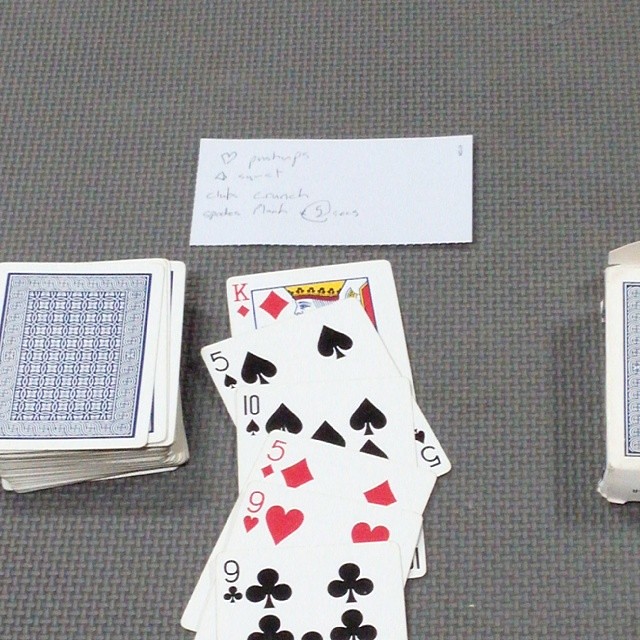The photo features a stack of rectangular playing cards arranged on a woven gray tablecloth. The cards' backs display a blue square adorned with small white stars, bordered by white. On the right, the edge of the box the cards came in is partially visible. In the center, several cards are spread out face-up in a somewhat loose arrangement. Notable among them are:

- The Nine of Clubs, which showcases a pattern of three-leaf clovers.
- The Nine of Hearts, marked by a red heart below the number and larger red hearts throughout the card.
- The Five of Diamonds, displaying red diamond shapes.
- The Ten of Spades, identified by spade symbols resembling upside-down hearts with attached stems.
- The King of Diamonds, which features a crowned man gazing forward beside a red diamond.

Above these cards, an additional white piece of paper with a heart and some text is visible, adding a slight personal touch to the arrangement.